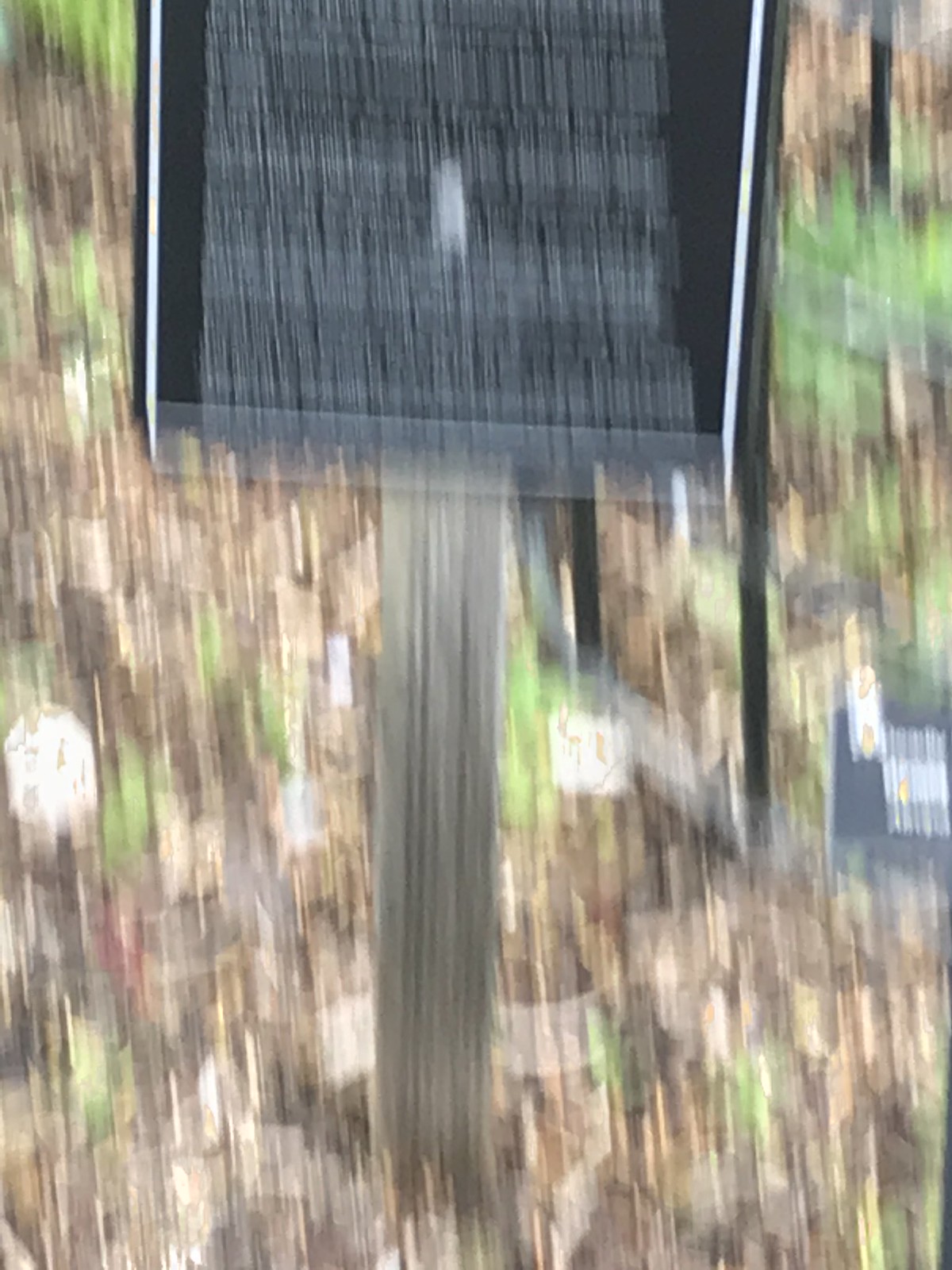The image in question is a highly blurred photograph, likely taken with a shaky camera, resulting in short, vertical, streaky lines across the picture. The main subject appears to be a black rectangular sign, mounted on a post. There's a consensus that the post could be brown wood or metallic, and the sign features some indecipherable white text or markings, possibly with a thin white border. The surroundings indicate an outdoor setting, with a mix of ground cover that includes dry leaves in shades of creamy, light, and dark brown, interspersed with patches of bright green grass. Additional blurred shapes in the background suggest there could be more posts or signs, some in black or dark brown with spots of white and yellow.